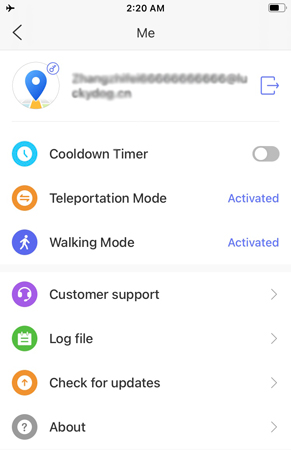The image appears to be a screenshot from a smartphone, specifically showing an app's settings interface. 

At the very top left corner is an airplane mode icon, signifying that the device might be in airplane mode. Centered at the top is the time, displayed as 2:20 AM, flanked on the right by a battery icon. Below the time, the text "Me" is displayed in black with a back arrow to the left of it, likely indicating a user profile or personal settings page. 

Under the "Me" label, there is a grayed-out email address that is so fuzzy it is unreadable. To the right of the email address is an icon, and to the left is a map pin icon, possibly indicating location settings or information.

The primary content in the middle of the screen consists of a series of options organized in rows, each accompanied by either slide buttons, the word "activated," or arrows. From top to bottom, the options are as follows:
1. "Cool-Down Timer" with a slide button, accompanied by a clock icon on a blue background.
2. "Teleportation Mode" marked as "Activated," with two arrows on an orange background.
3. "Walking Mode" also marked as "Activated," with a walking person icon on a blue background.
4. "Customer Support" with an arrow, featuring a headset icon on a purple background.
5. "Log File" with an arrow, accompanied by a notebook icon on a green background.
6. "Check for Updates" with an arrow, displayed with an upload icon on an orange background.
7. "About" with an arrow, with a question mark icon on a gray background.

This detailed layout provides a clear overview of the various settings and functionalities available within the app.